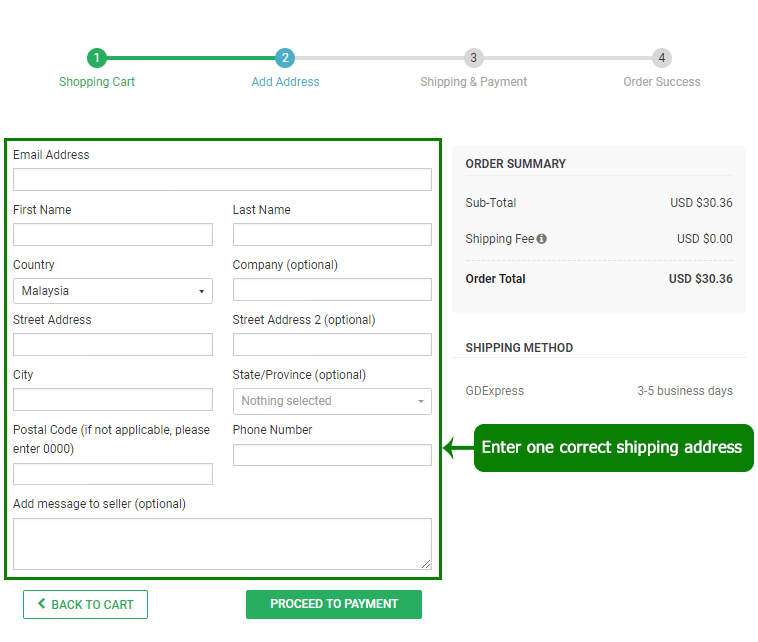Here is a screenshot of an online order page, meticulously organized into four sequential steps displayed at the top: 1. Shopping Cart, 2. Add Address, 3. Shipping and Payment, and 4. Order Success. Each step is designated by an evenly spaced number along a continuous line, creating a clear visual guide for the user.

Dominating the left side of the page is a large green rectangle, within which are several text fields requiring user input. The fields include: Email Address, First Name, Last Name, Country (preset to Malaysia), Company, Street Address, Street Address 2 (optional), City, State/Province (optional), Postal Code (with instructions to enter 000 if not applicable), Phone Number, and Add Message to Seller (optional). Directly beneath this green section, two distinct buttons are available for navigation: one to return to the Cart, and another labeled "Proceed to Payment" for moving forward with the order.

On the right-hand side, an order summary is presented within a light gray rectangle. This summary details the Subtotal as USD 30.36, Shipping Fee as USD 0.00, and consequently, the Order Total also as USD 30.36. Below the summary, the Shipping Method is noted, specifying "GD Express 3-5 Business Days." At the bottom of the page, another green rectangle underscores the importance of accuracy by directing the user to "Enter One Correct Shipping Address," ensuring the delivery details are meticulously correct.